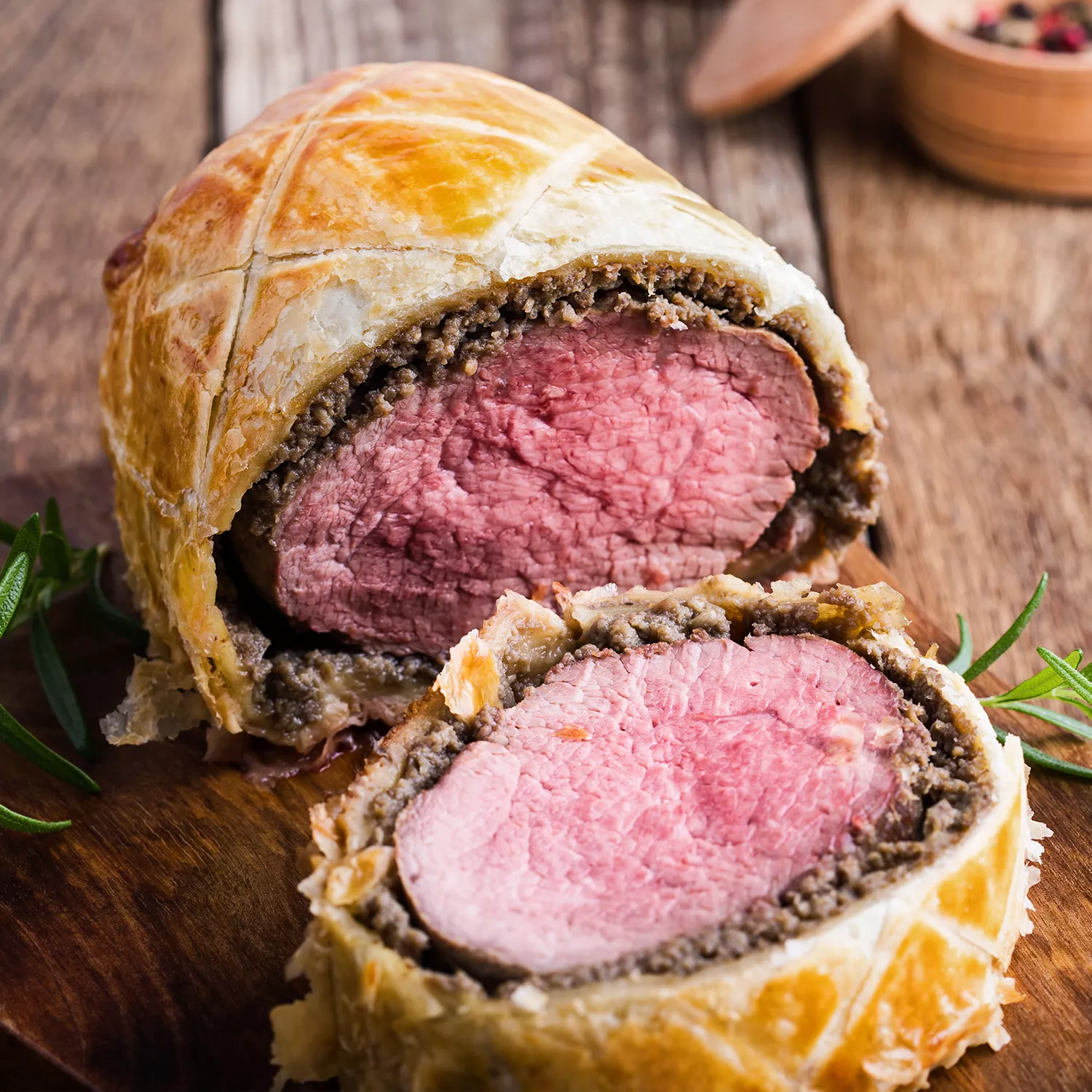In this image, we observe a beautifully detailed scene centered around a succulent slice of beef wellington placed on a wooden chopping board. The beef wellington, a savory pastry-wrapped dish, reveals its impressive layers upon being cut—an enticing pink and juicy beef fillet nestled in a flavorful brown mushroom duxelles, all encased within a golden-brown, flaky pastry crust. The brown chopping board showcases fine lines and grooves, enhancing the rustic appeal of the setup. Surrounding the beef wellington are sprigs of fresh rosemary adding a touch of green. The top right corner of the image features an orange bowl with its lid ajar, hinting at additional ingredients or accompaniments, further enriching the culinary scene. The composition of the photo emphasizes the exquisiteness of the beef wellington while providing a warm and inviting ambiance with its earthy tones and carefully arranged elements.